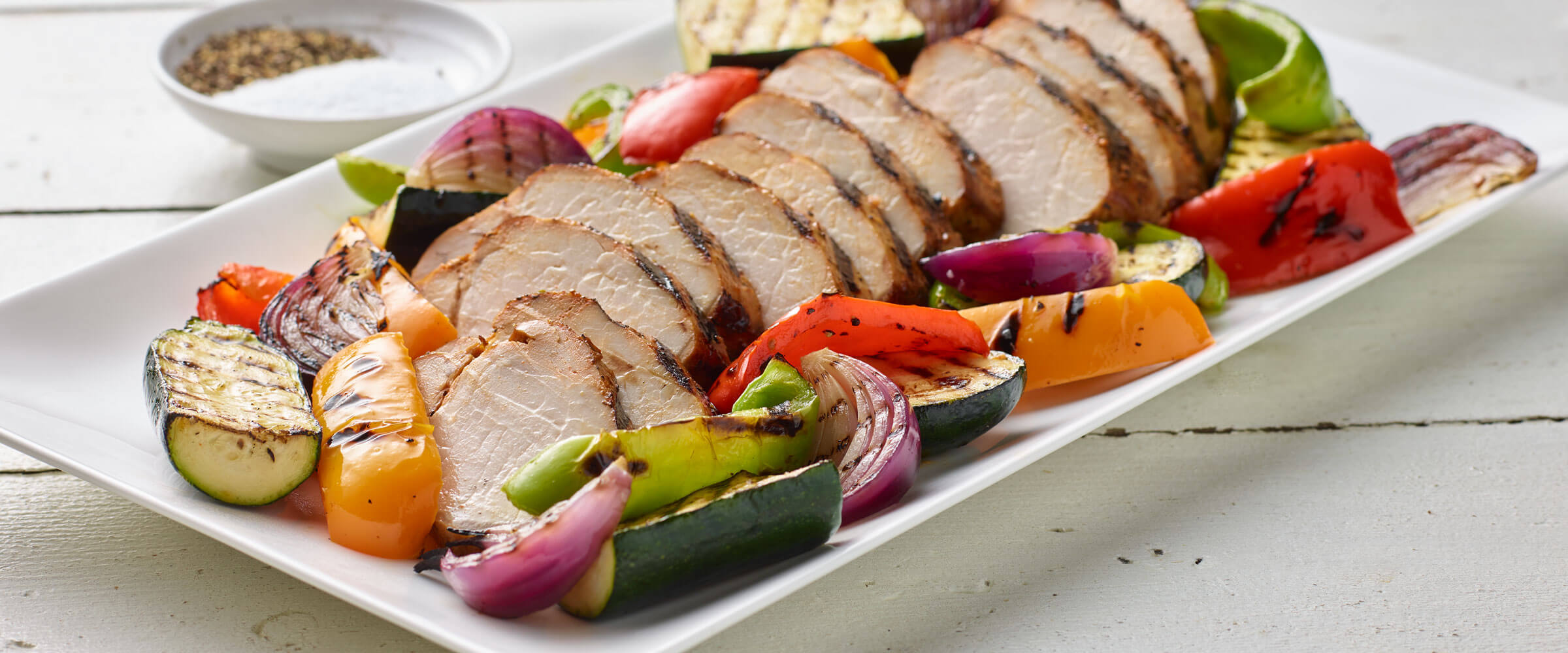The image showcases a beautifully arranged, nutritious meal set on a white Summerswood painted wooden table, bathed in daylight, suggesting an outdoor gathering like a barbecue or picnic. On a clean white platter, perfectly sliced, charbroiled chicken (or possibly pork) is surrounded by an array of vibrant, grilled vegetables, including zucchini, red, yellow, and green bell peppers, and red onions. Accompanying the dish is a small bowl placed to the left, likely containing salt and pepper, and a light vinaigrette sauce on the right, adding to the summery, light, and healthy appeal of the meal.